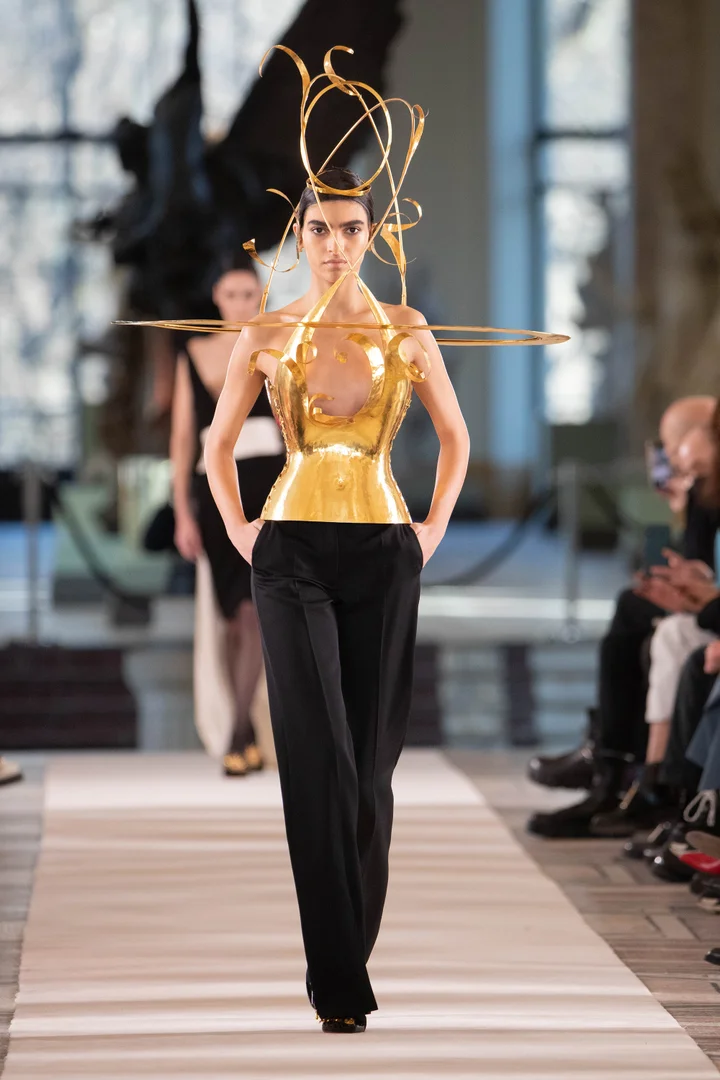This color photograph captures the moment at a high-fashion runway show where a model strides confidently toward the camera on a ground-level catwalk, flanked by an audience seated to the right, their legs casually crossed or flat on the floor. The model, a white woman with short, black hair and thick eyebrows, wears black dress pants and black shoes, with her hands partially tucked into her pockets up to the last knuckle. Her striking golden top, a halter style that leaves her shoulders bare, features intricate, thin gold swirls and wisps extending around her body. A prominent circular gold ring sits at her shoulder level, around which rods project and curve upwards and outwards like decorative leaves. The runway is a beige carpet, and in the background, another model awaits her turn, dressed in more conventional attire. The scene is set against a backdrop featuring a large black sculpture, windows, and a platform with a staircase leading up to it, adding to the high-fashion ambiance.